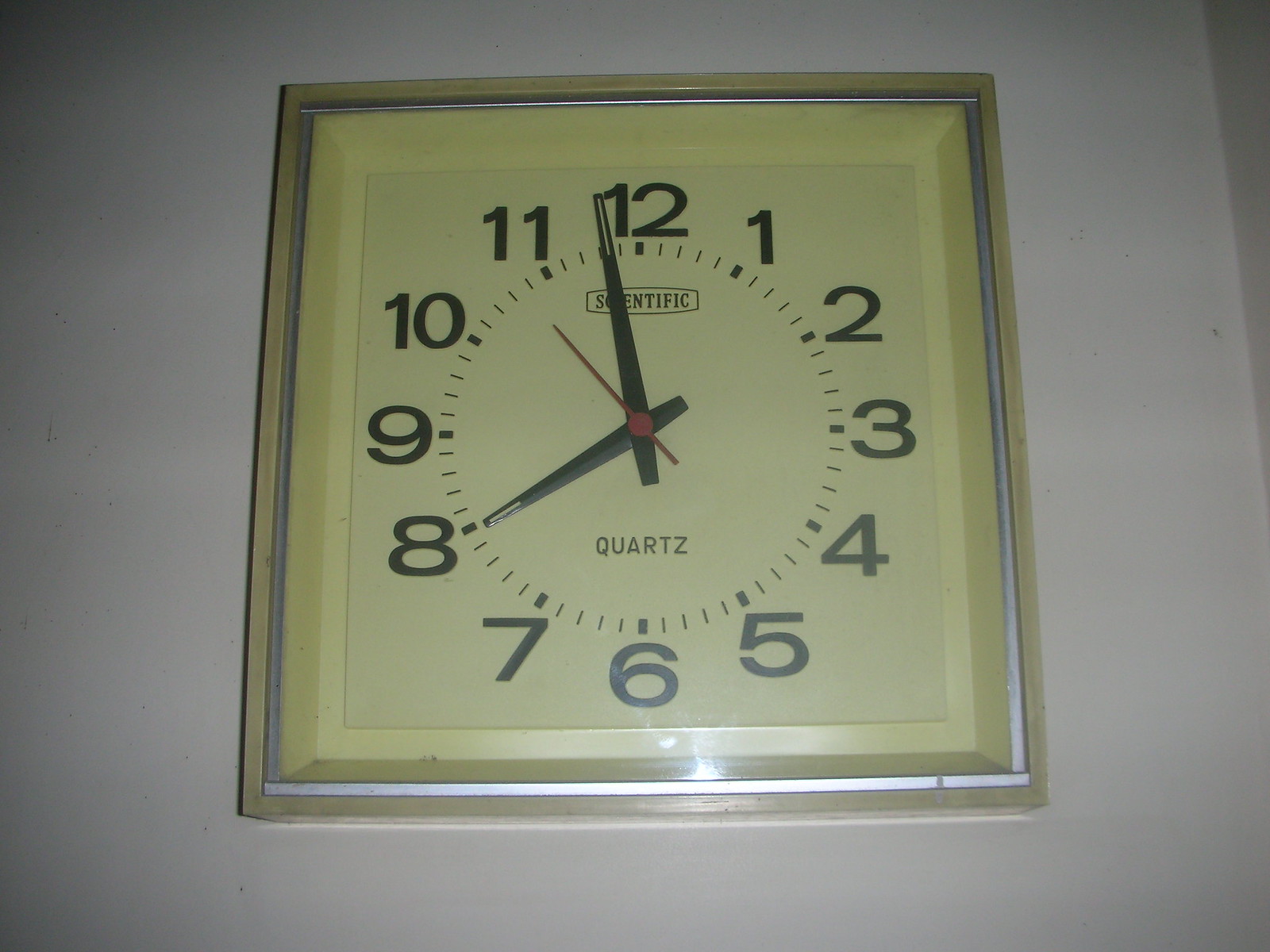This close-up photograph captures a square-shaped clock with a sleek silver border, prominently displayed against a white wall. The clock face features an off-white background with bold black numbers and a distinct black and red dial. At the top of the clock face, the word "Scientific" is prominently displayed, while "Quartz" is inscribed near the bottom. The clock reads 7:58, and a small reflection from the camera flash can be seen near the bottom center of the clock face, adding an additional layer of detail to the image.